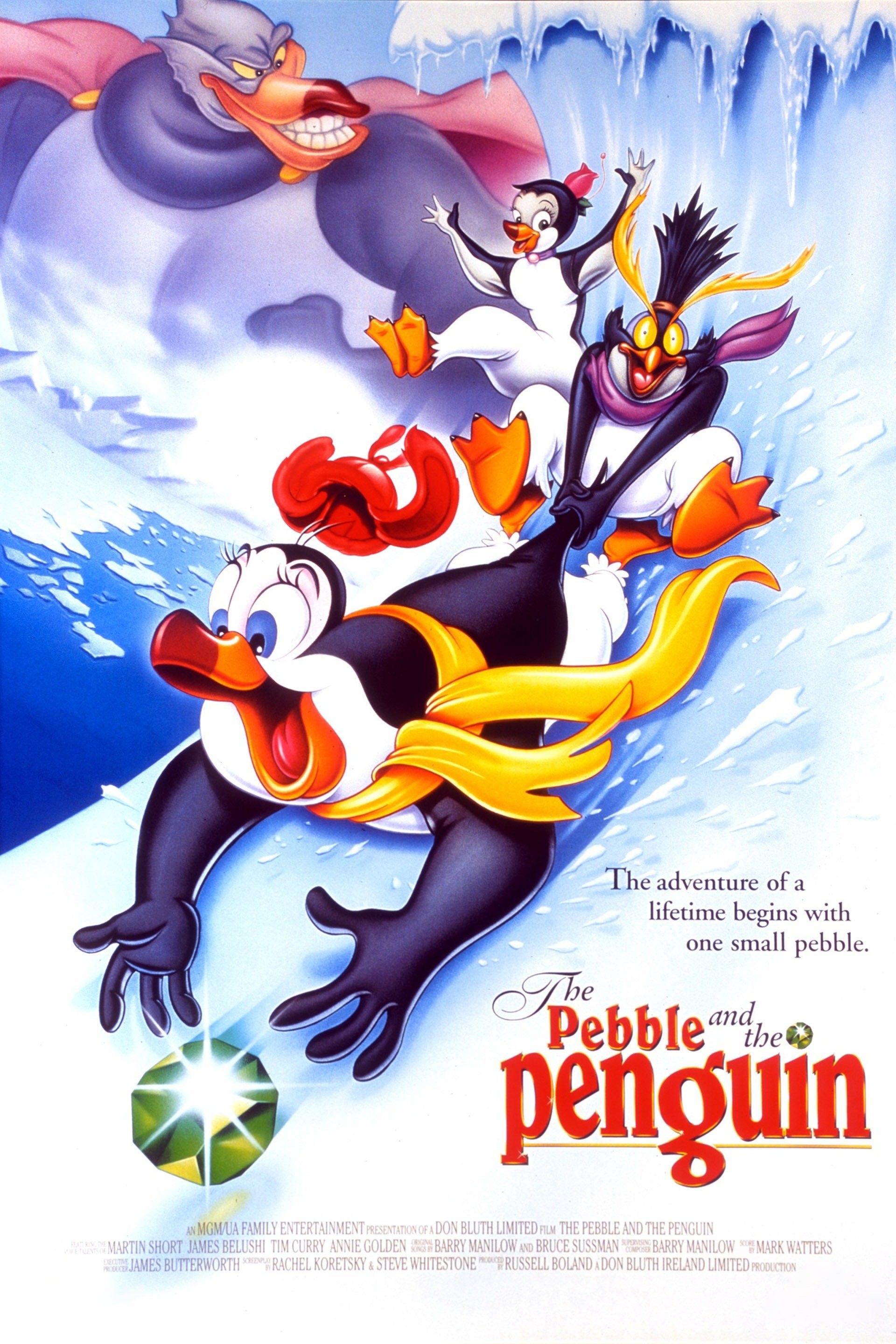This vibrant and colorful movie poster, titled "The Pebble and the Penguin," features an exciting scene set against a pale blue background. Bold red letters spell out "Pebble Penguin" in the bottom right corner, surrounded by smaller black text completing the full title as "The Pebble and the Penguin." Above this, the tagline reads, "The adventure of a lifetime begins with one small pebble." 

Central to the illustration are three animated penguins joyfully sliding down a snowy or icy hill, appearing as though they are riding a wave. The foremost penguin, clad in a yellow scarf with an agape red and orange beak, reaches excitedly for a large emerald with a radiant white star at its center. Directly behind, another penguin, similarly colored and adorned with a magenta scarf, clutches the tail of their friend, attempting to slow their descent. The third penguin, more white than black and sporting a red bow on its head, follows suit with orange feet and an orange face, completing the line.

Bright, vivid colors, including yellows, reds, oranges, and blues, enrich the scene, adding a sense of vibrant motion and energy. In the background, a large, menacing monster with purple skin, a pink cape, and prominent teeth looms ominously, chasing after the trio. The backdrop features earth-like hues of blue and white, reminiscent of satellite imagery, enhancing the sense of adventure and urgency in this captivating animated escapade.